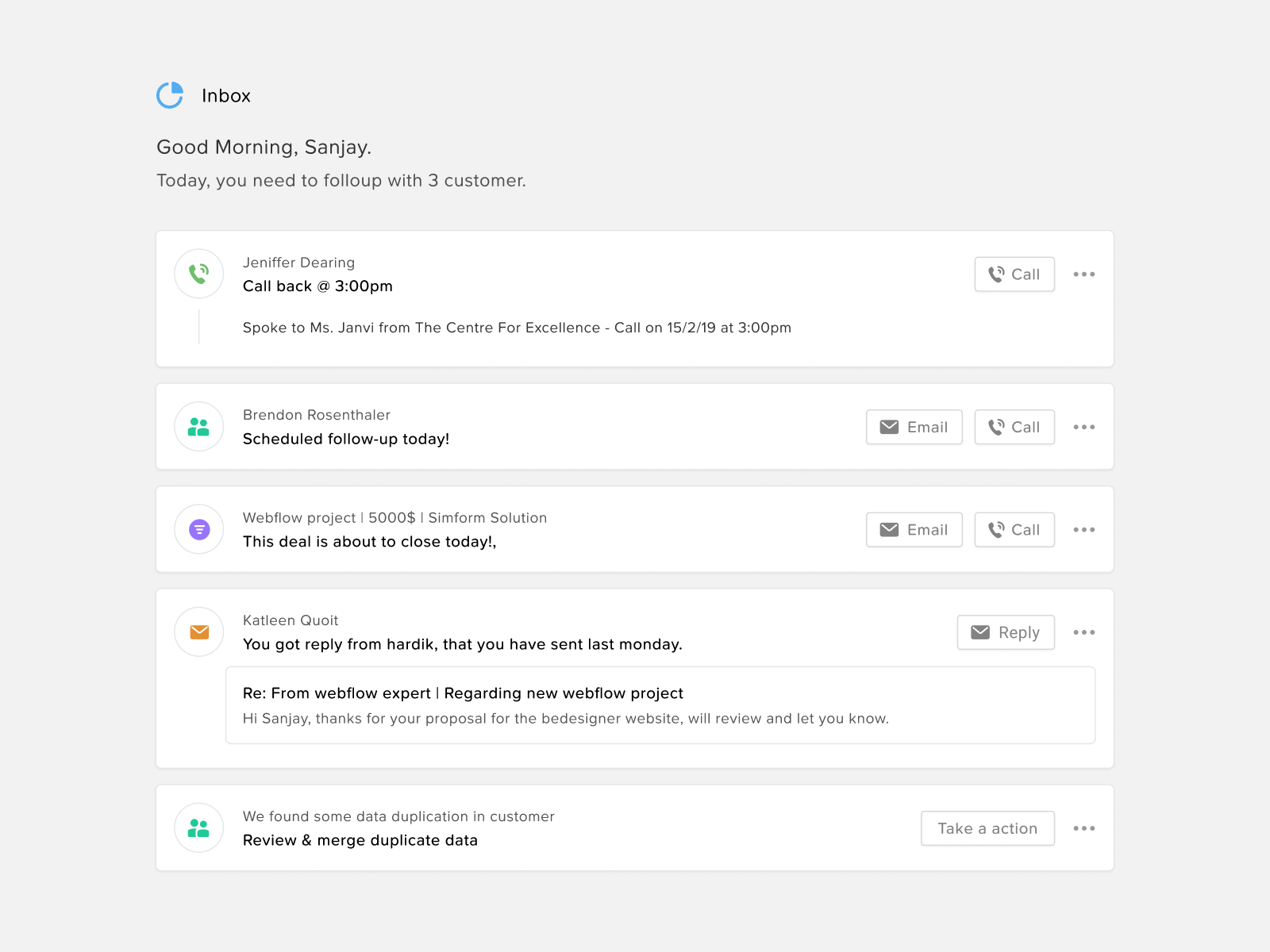In the center of a light gray-colored background box, the upper left corner features a blue circle icon with the word "Inbox" written in black. Below this, the text reads, "Good morning Sanjay, today you need to follow up with three customers," although there is a typo with "follow-up" spelled as "follou up."

Beneath this introduction, a series of white boxes detail various tasks:

1. The first box contains a call icon on the left and the text "Jennifer Deering: Call back at 3 p.m." To the right of this text, there is a call button.
2. The second box features a group icon with the text "Brendan Rosen hire: Schedule follow-up today." Next to this, on the right, there are email and call buttons.
3. The third box displays a purple icon with the text "Web Flow Project 5000: This deal is about to close today." To the right, there are email and call buttons.
4. The fourth box includes an email icon and the text "Kathleen Wait: You got a reply from Hardik that you sent last Monday." Adjacent to this text, there is a reply button.
5. The fifth and final box showcases a group icon with the text "Review and merge duplicate data," followed by a take action button on the right side.